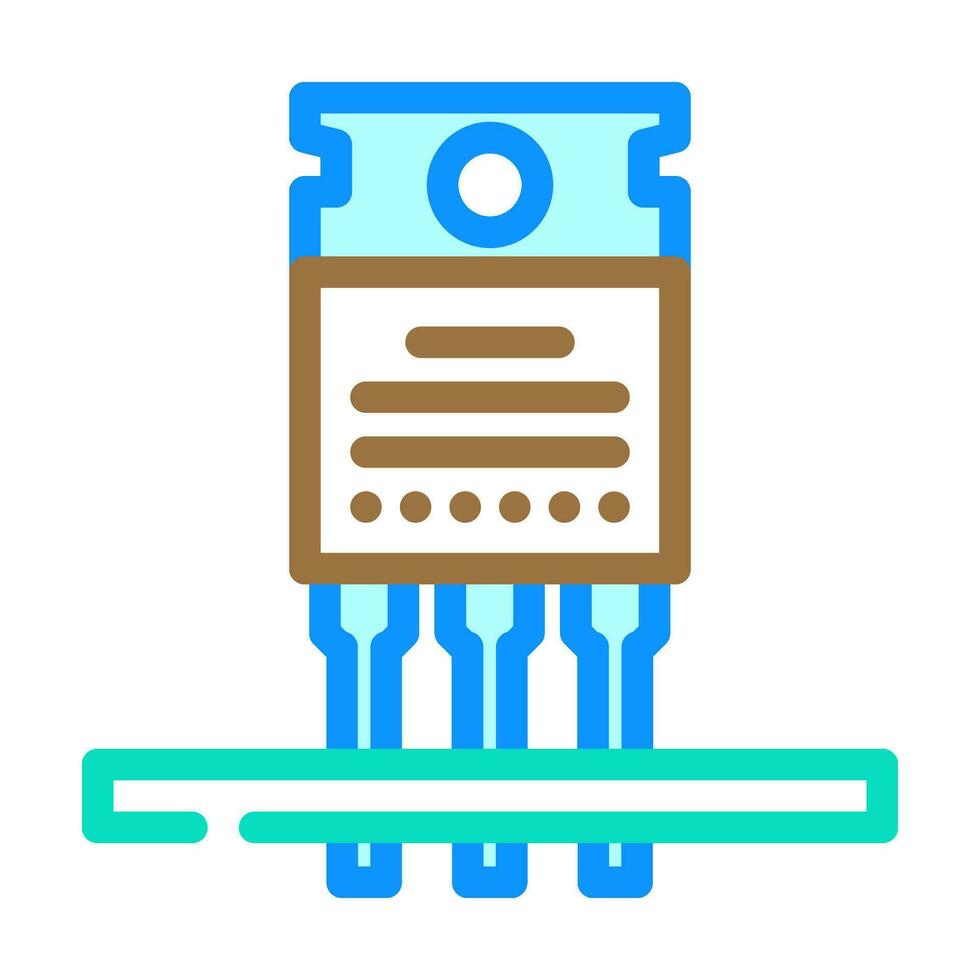The image features a detailed icon, depicted on a solid white background, resembling a microchip or circuit board. The central element is a brown square with three horizontal lines and several brown dots inside, evoking the layered complexity of electronic components. Above the square, a blue shape, reminiscent of a razor blade, sports an empty circle in its center. The structure is supported by three downward-pointing prongs outlined in blue, filled with a lighter blue shade. At the base, a light green outlined rectangle, similar to an incomplete paperclip, anchors the design. The entire composition is marked by its use of thick lines and vibrant colors, suggesting it was created using digital tools like Adobe Illustrator or Microsoft Paint.